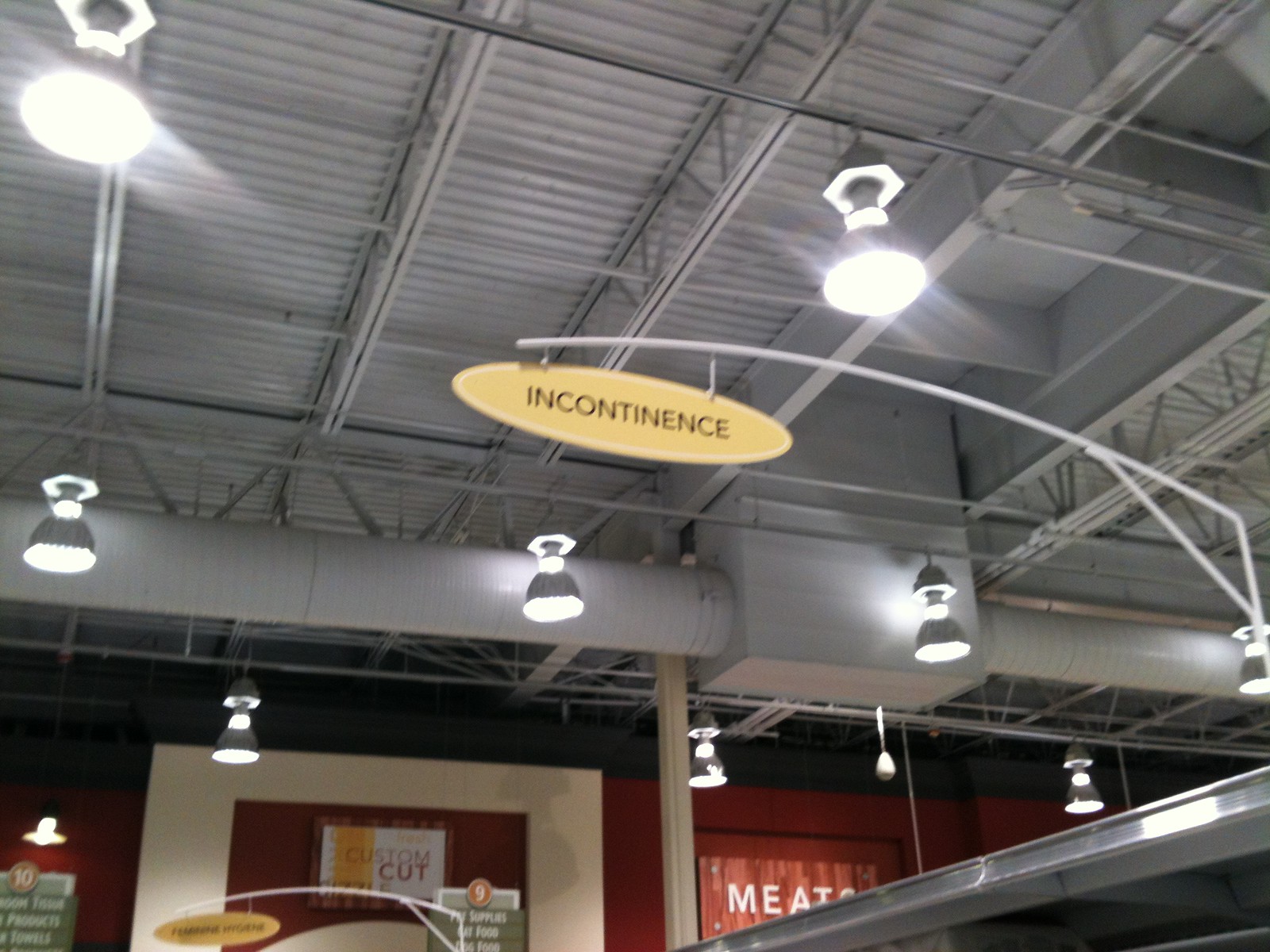The photograph captures the interior of a large, industrial-looking grocery store or meat market, viewed from an angle that emphasizes the ceiling and the middle of the building. Dominating the scene is a grey metal ceiling adorned with an intricate network of ducting and pipes, along with numerous hanging lights that illuminate the space. 

At the center of the image, a long white pole extends from the right side, supporting a puzzling yellow sign that reads "incontinence." This sign seems out of place in the grocery store setting. Below this sign, the top part of a red wall can be seen, featuring various signs. One sign prominently reads "custom-cut," while another partially visible sign indicates the meat section with the word "meats." There are also some aisle indicators, specifically for aisles number nine and ten. 

The overall ambiance of the photograph conveys an industrial aesthetic, characterized by its functional design geared towards utility, yet interrupted by the curious signage.